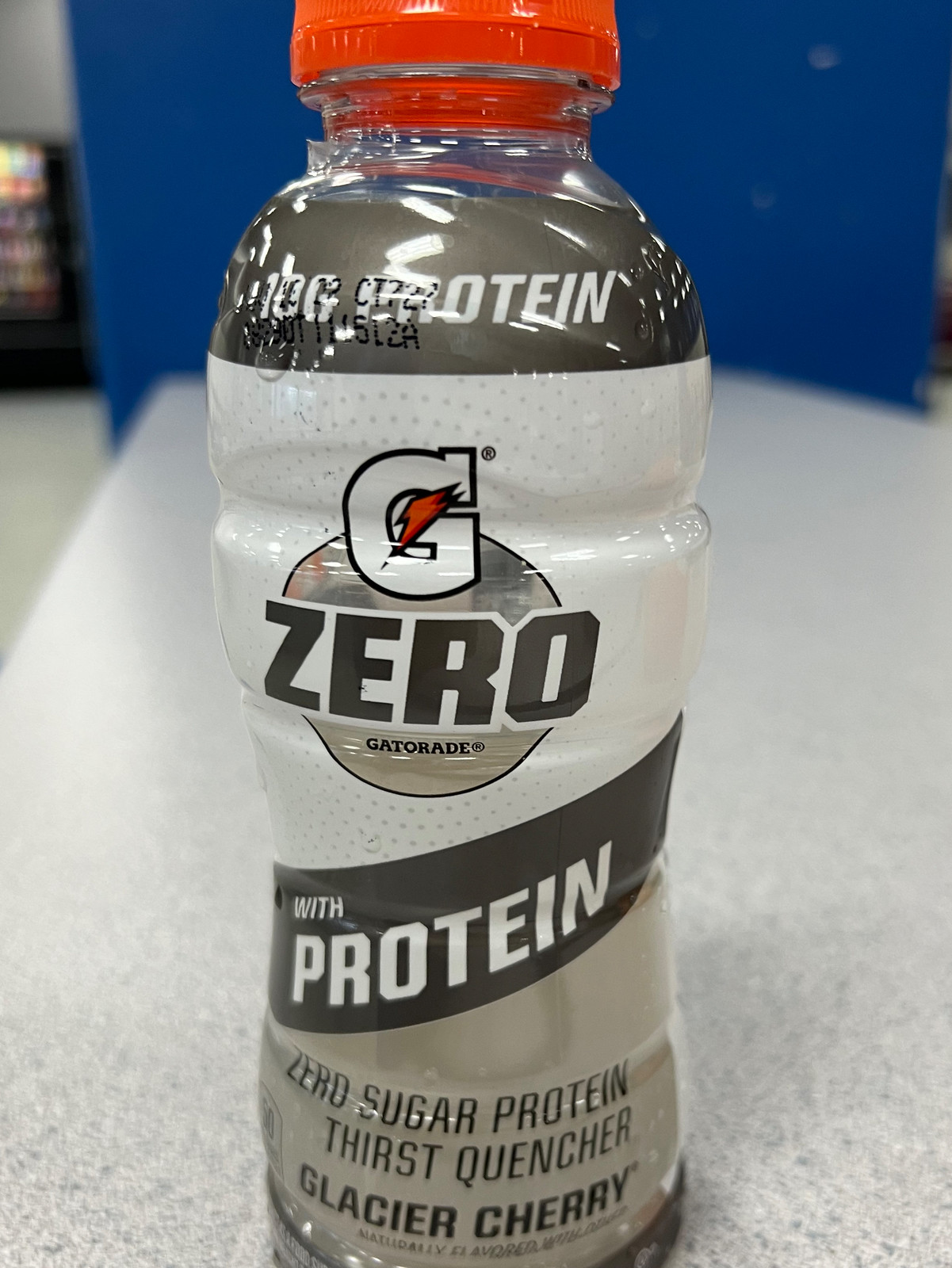This is a close-up, vertical, color photograph of a Gatorade Zero bottle, prominently featuring its detailed label and surroundings. The clear plastic bottle, capped with an orange top and ring around the neck, has a full-wrap label in a combination of white, black, and tan, with accents of orange and hints of red. At the top of the label, in large white block letters outlined in black, is the letter 'G' with an orange lightning bolt through the middle. Beneath this, in black text, it states "ZERO" in a circular design bordered by a black ring, followed by smaller capital letters spelling "GATORADE."

Across the label, a black banner runs diagonally from the bottom left to the middle right, emblazoned with "WITH PROTEIN" in white capital letters. Below this, in black capital letters, it reads "ZERO SUGAR PROTEIN THIRST QUENCHER." At the bottom of the label, the flavor "GLACIER CHERRY," which is naturally flavored, is prominently displayed in bold black text. Additionally, the label specifies "10G PROTEIN" at the top, reinforcing the drink's protein content.

The bottle, which appears unopened and contains no visible red liquid, is positioned on a white and gray mottled counter, casting a small shadow to the right. Behind the bottle, a bright blue wall provides a vibrant backdrop. There is also some blurred, unreadable information in the bottle's upper left corner.